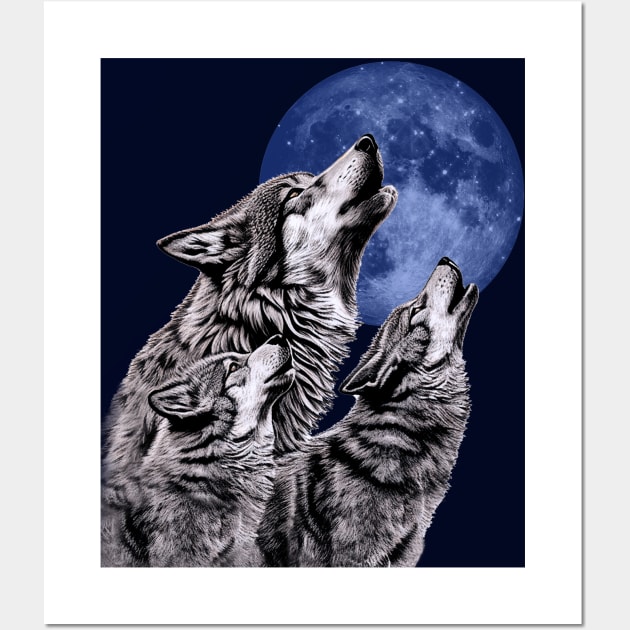The image is a detailed close-up of an art print featuring three realistically depicted wolves howling at a bluish-white, cratered moon, set against a dark navy background. The artwork has a white rectangular border, with gray bars on the left and right sides, creating a square framing. The wolves, rendered in black and white, show intricate details in their fur, ears, eyes, noses, and mouths. Arranged from the bottom left corner, their heads are lifted towards the upper right, where the moon is placed, their ears pointed back. The wolves appear to be of different sizes, suggesting possibly a parent with two offspring. Their thick fur has dark areas along the neck and under the chin, adding to the lifelike texture. The moon, detailed with craters and subtle sparkles, enhances the mystical ambiance of the scene.